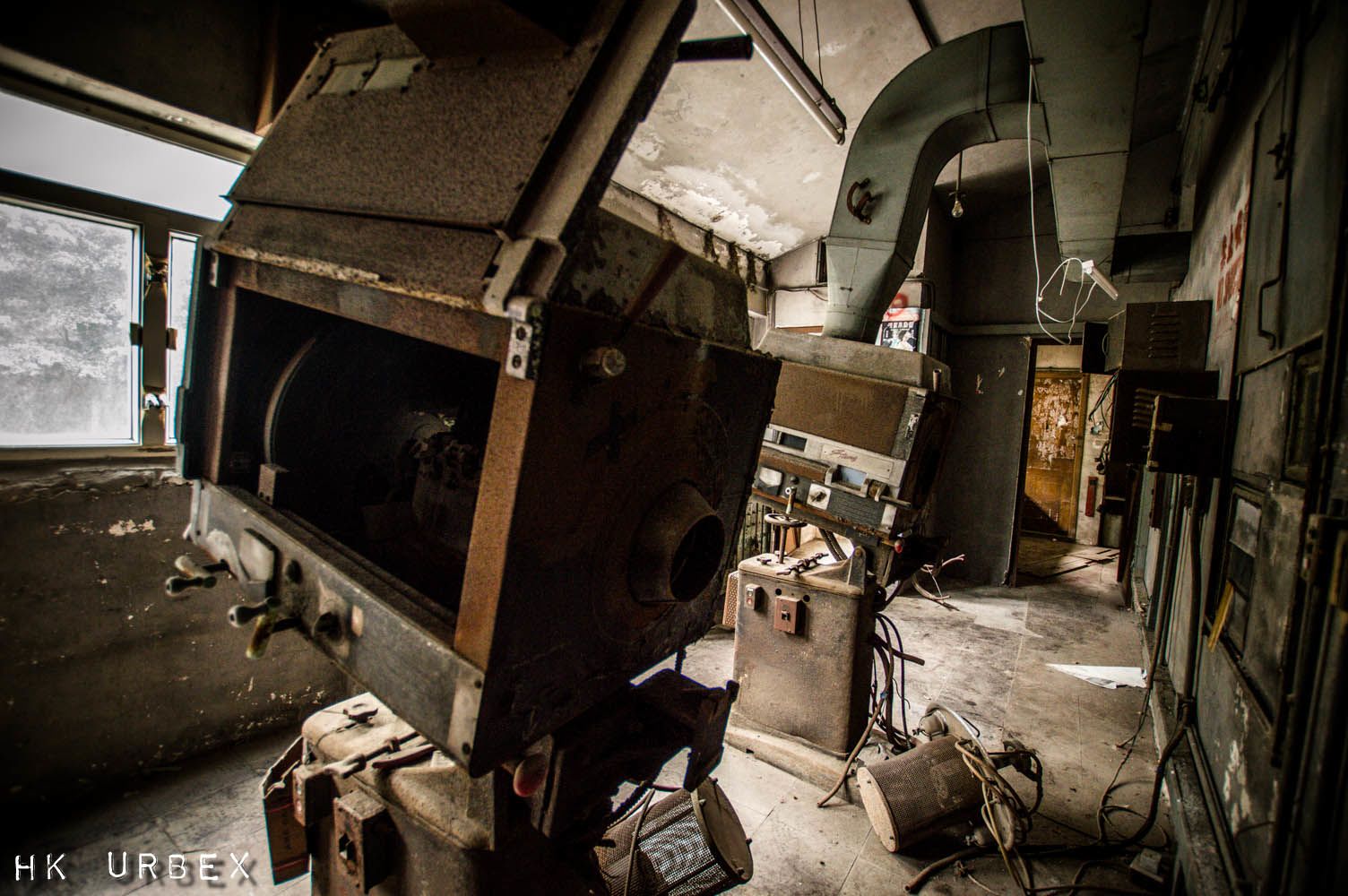The photograph, taken in landscape orientation, captures a room within an old, dilapidated factory. The scene is filled with signs of disuse and decay, featuring numerous rusty surfaces and accumulated grime. Dominating the foreground on the left-hand side is a large metal structure, possibly an old industrial oven, equipped with various dials and levers. Behind this apparatus stands another similar piece of equipment, distinguishable by a prominent exhaust pipe extending into the ceiling. 

Windows on the left wall allow a small amount of natural light to filter into the otherwise dimly lit space, revealing hanging, disconnected wires and several filter cages carelessly strewn across the floor. On the right-hand side, a door leads to another area of the factory, inviting curiosity about what lies beyond in this abandoned industrial labyrinth.